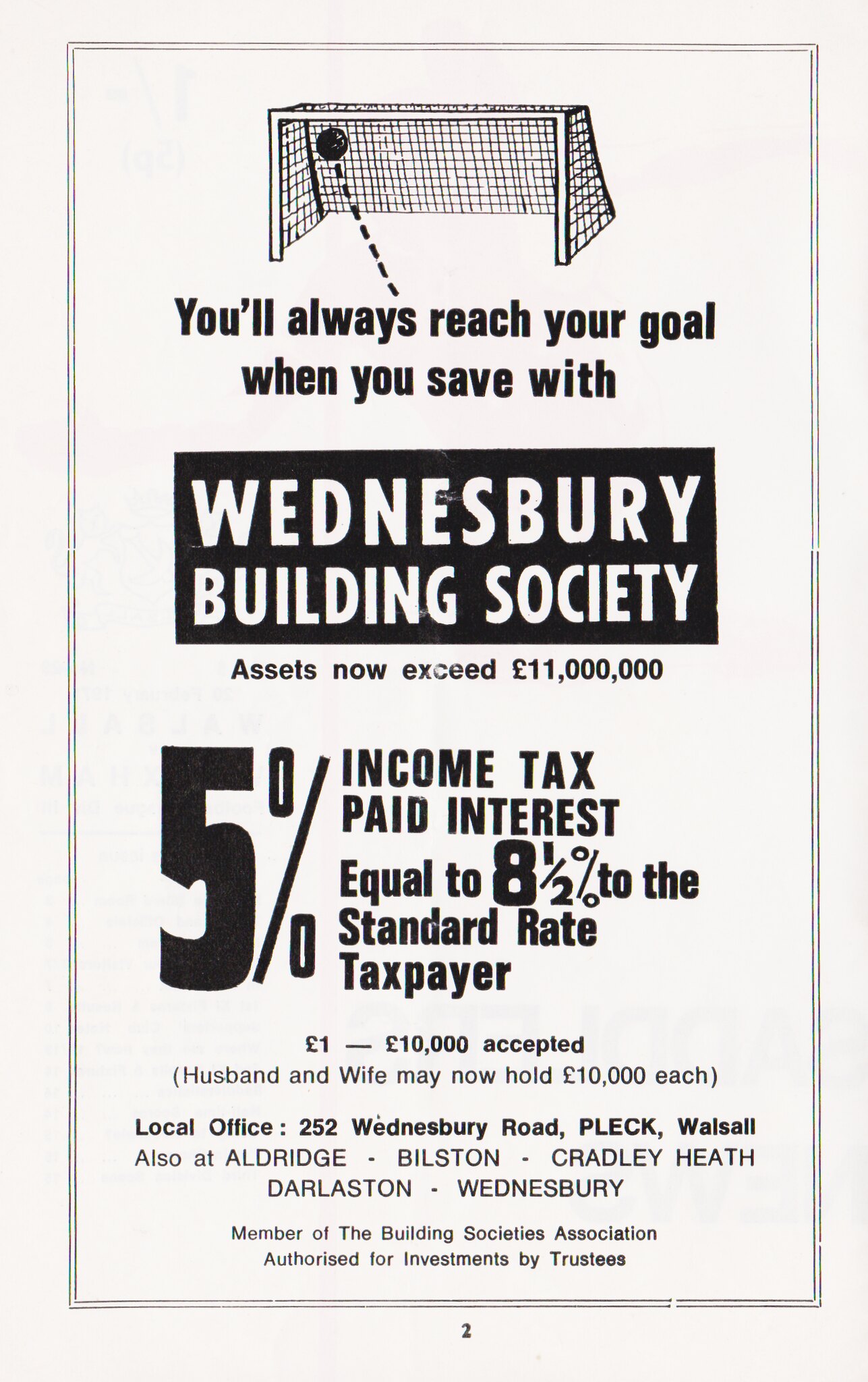This black-and-white print advertisement, likely from a newspaper, prominently features a simplistic graphic of a soccer goal with a soccer ball scoring, symbolizing the potential success of saving. Highlighted by a black border on white paper, the ad declares in bold text, "You'll always reach your goal when you save with Wednesbury Building Society." It proudly announces that the society's assets have now exceeded 11 million pounds. The ad details that savers can earn a 5% income tax-paid interest, which equates to an 8.5% rate for standard taxpayers. Notably, it mentions that deposits ranging from one pound to 10,000 pounds are accepted and that husbands and wives can now each hold up to 10,000 pounds separately. Moreover, it lists various branch locations, including the local office at 252 Wednesbury Road, Plek, Walsall, and additional branches in Aldridge, Bilston, Cradley Heath, Darleston, and Wednesbury. The advertisement underlines its legitimacy as a member of the Building Societies Association and is authorized for trustee investments.